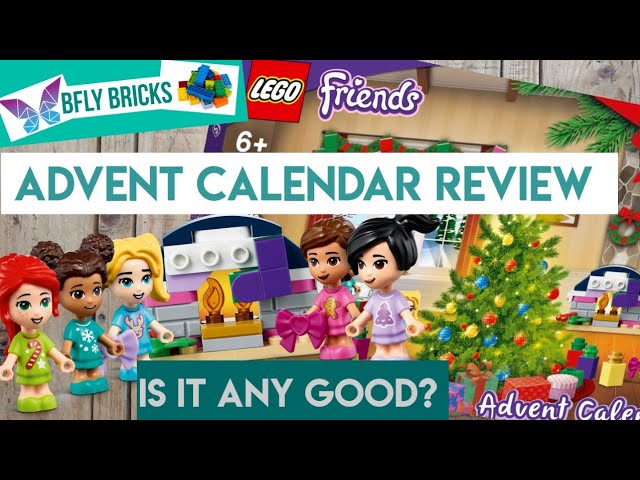The image displays an advertisement for LEGO Friends, specifically for the "Butterfly Bricks" set, shortened to "B-F-L-Y, Beefly Bricks." At the top left, a purple and blue butterfly graphic is positioned next to the words “Beefly Bricks” in green, capitalized text, set against a white background. To the right, there’s a small pile of LEGO pieces next to the iconic LEGO logo in white on a red background. Adjacent to this, the word “Friends” is styled in a script font, also in white on a purple background, with heart-dotted "i"s. Below, a white banner with green, all-caps text reads, “Advent Calendar Review,” and at the very bottom, over a green background, is the white, all-caps text, “Is it any good?” To the right of this, the word “Advent” appears partially, with only "C-A-L-E" visible in a white script font outlined in purple.

In the central part of the image, a row of LEGO figures presents various female characters: three figures on the left, two in the center, and three on the bottom, with the left and bottom figures facing towards those in the center. These characters include a redhead, a black girl, and a blonde girl with pigtails among others. On the right side, a brown-haired girl and an Asian or Filipino girl with short black hair styled in a bob are visible. The scene features a Christmas tree with LEGO presents around it, suggesting a festive, holiday theme.

This composite image appears somewhat assembled from various sources and is set against a gray wood panel background, which adds to the collage-like appearance.